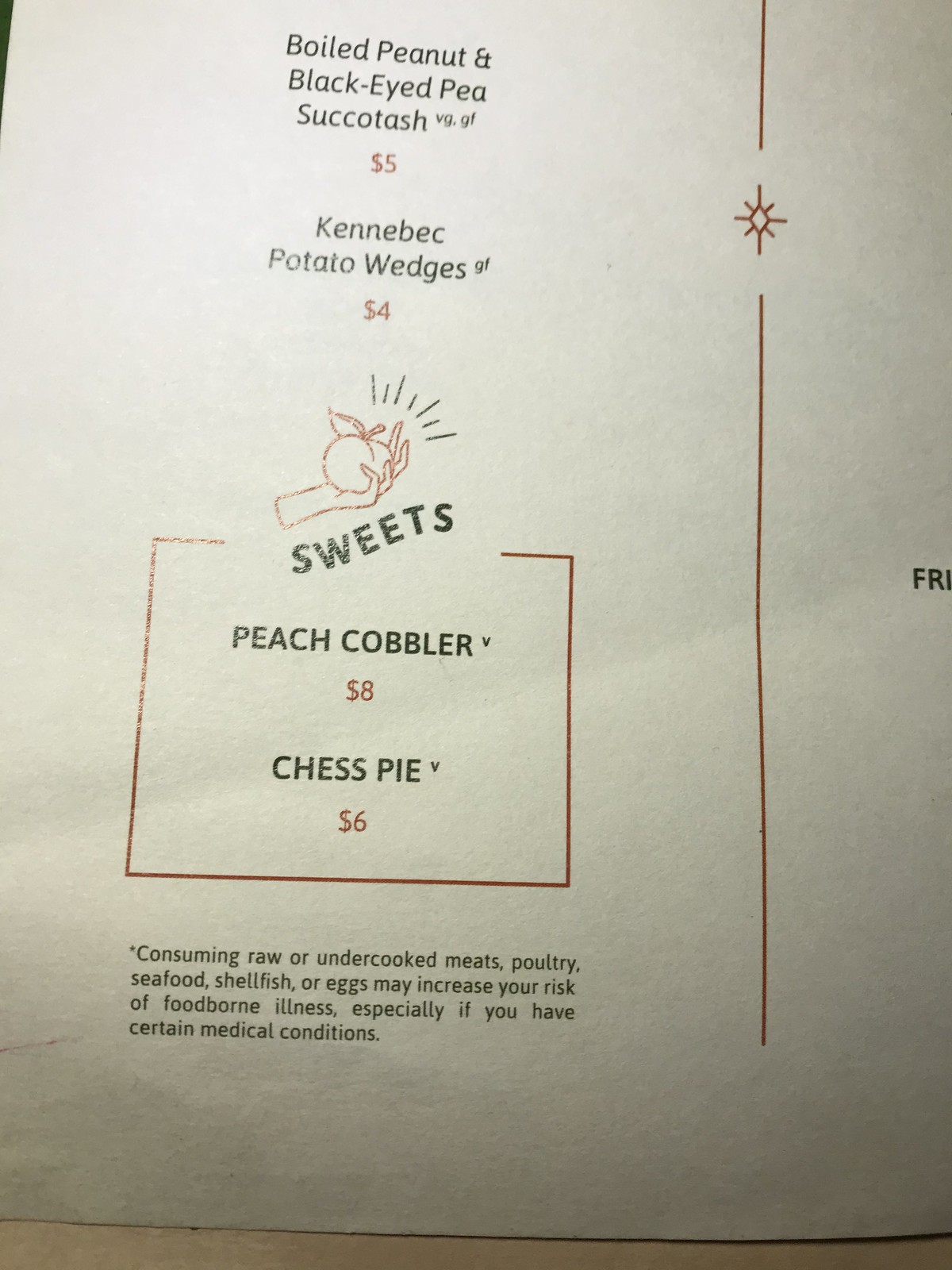The image captures the lower left-hand corner of a restaurant menu. The top item listed is "Boiled Peanut and Black Eye Pea Succotash," denoted as both vegetarian and gluten-free (VG.GF) and priced at $5. Beneath that, there’s "Candy Back Potato Wedges," also labeled gluten-free and costing $4. The menu section titled "Sweets" features a hand holding a peach image. Under "Sweets," the menu lists "Peach Cobbler" at $8 and "Chess Pie" at $6. At the bottom, a small asterisked disclaimer advises that consuming raw or undercooked meats, poultry, seafood, shellfish, or eggs may pose health risks, particularly for individuals with certain medical conditions.